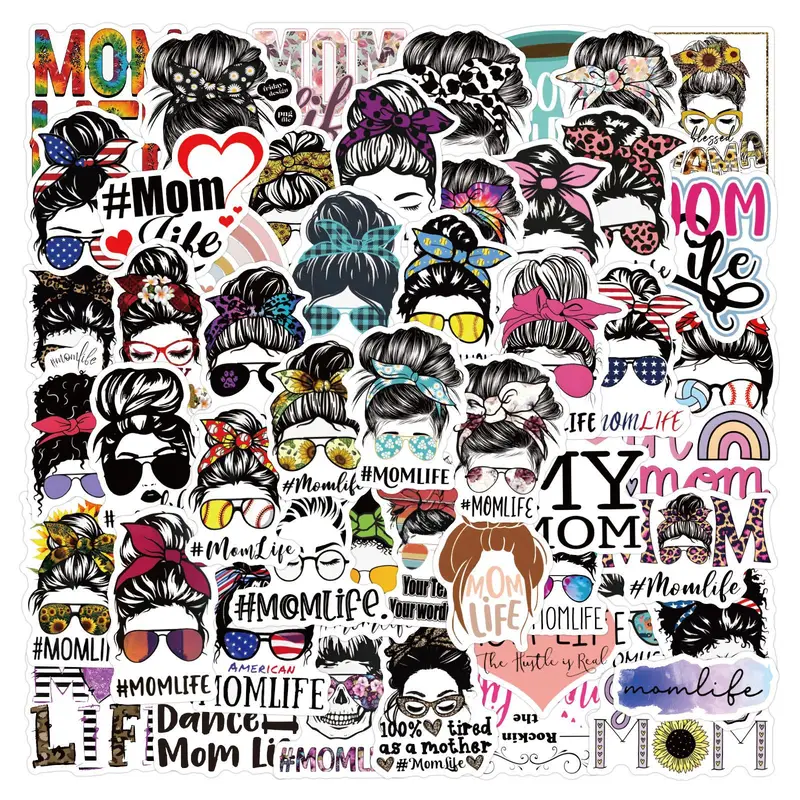The image is a vibrant and colorful square collage art piece, intricately covered with numerous overlapping die-cut images, resembling scrapbooking stickers. Dominating the collage are repetitive yet slightly varied cartoon-like depictions of women's faces wearing different styles of sunglasses – some reflecting sunflowers, with others featuring patterns like gingham check, or even patriotic themes. Most of these women have their hair gathered up into top buns, often tied with colorful bandanas, scarves, or floral wraps. Embedded among these images are various hashtags and phrases such as "Mom Life" and "Hashtag Mom Life," repeated in different scripts and vivid colors. Phrases like "Dance Mom 100%," "Love tired as a mother," and "Rockin' the life" accentuate the mom-centric theme. Scattered throughout are bright elements like hearts, rainbows, and sunflowers, all contributing to the lively, scrapbook-esque theme of the graphic design. The collage boasts a palette of diverse colors including purples, blues, pinks, reds, yellows, and greens, creating a visually captivating and celebratory representation of "mom life."